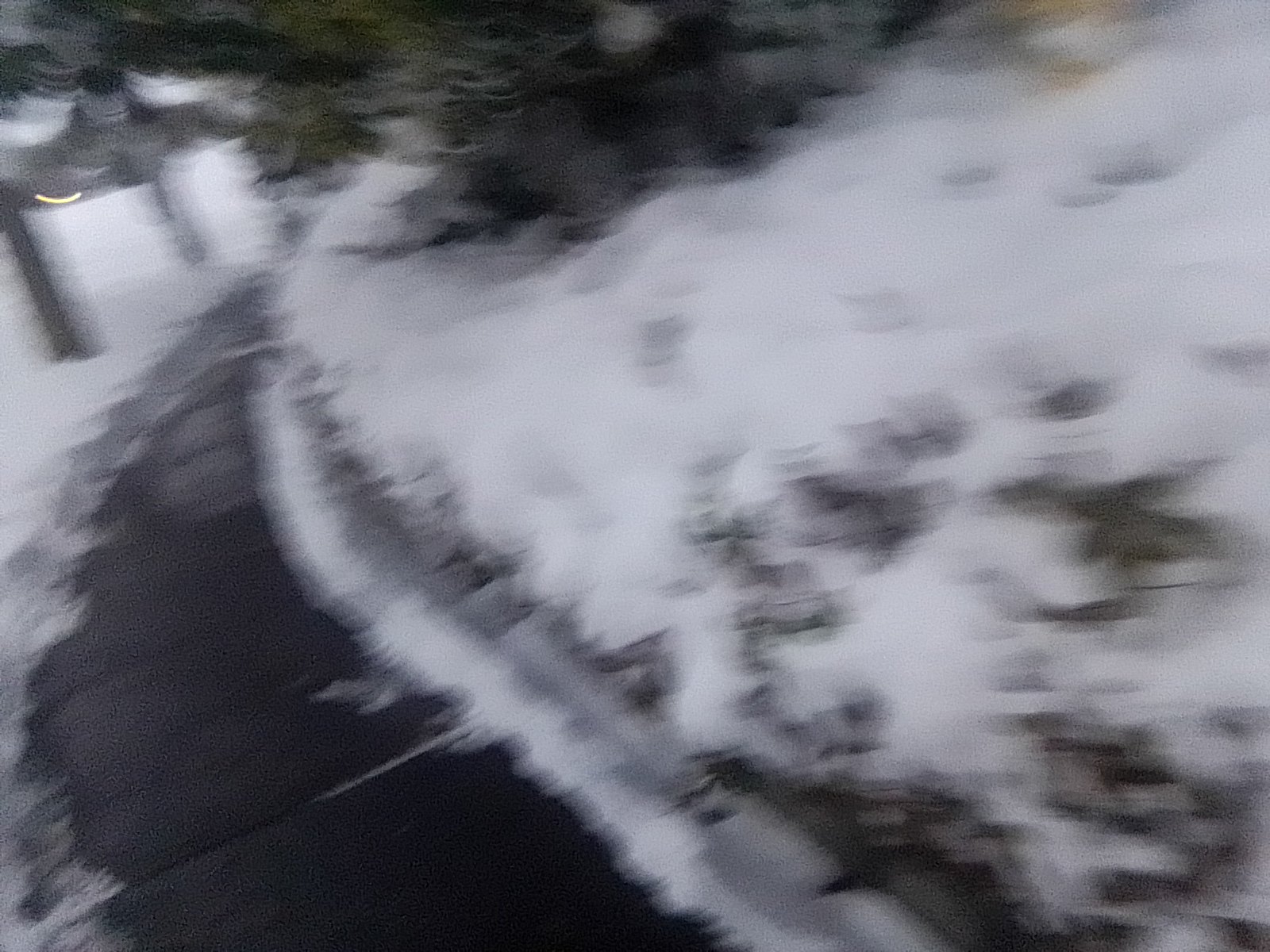This photograph, though very blurry and out-of-focus, captures a winter scene marked by a dark grey sidewalk curving from the bottom center to the upper center, veering towards the left. The sidewalk is largely cleared of snow, contrasting against the surrounding white, snow-covered landscape. To the left of the sidewalk, there are white objects, possibly trash cans, standing upright amidst the dense snow. The camera angle is slightly canted, offering a view downwards toward a snow-covered lawn and adjacent houses or privacy fences, also white. A tree, or some type of plant, is visible at the upper top center of the image, and there is light reflecting or illuminating from the upper left corner, suggesting either twilight or a late evening. The predominant colors in this image are grey, white, and green. There's no text visible, enhancing the focus on the serene, wintry outdoor scene.